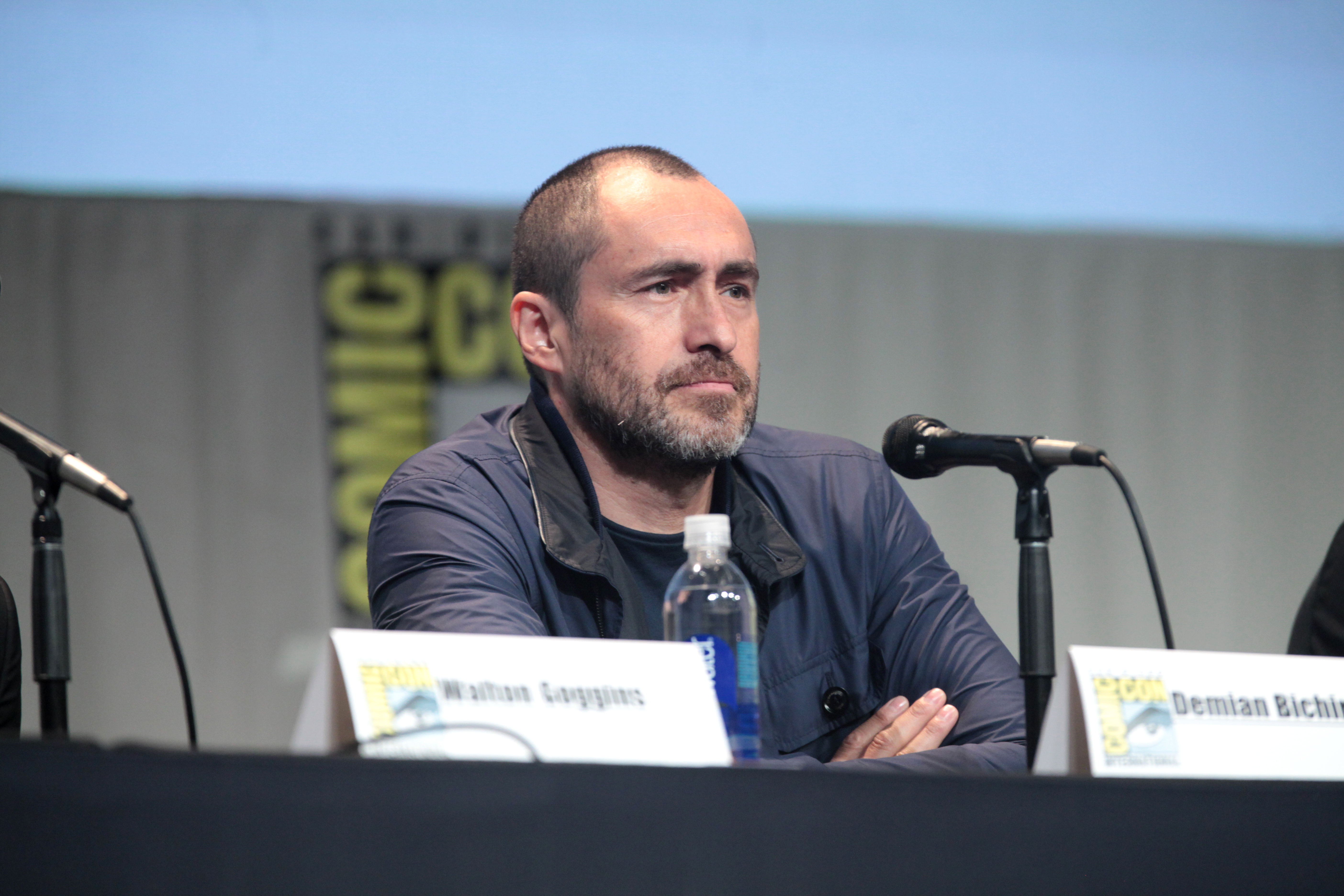The image depicts an indoor event, likely Comic-Con, indicated by a golden "Comic-Con" logo on the gray curtain in the background. The setting resembles a press conference with a long, gray table spanning the bottom one-sixth of the photograph. Two microphones on stands are placed at each end of the table, and in front of them are white name cards with black letters. The name on the right card reads "Demian Bichir." The man associated with this name card appears to be an actor, identifiable by his close-cropped dark brown hair, light beard, and mustache with gray at the chin. He is wearing a long-sleeved blue jacket over a blue sweater and has his arms folded on the table. There is also a water bottle in front of him. The table is covered with a black tablecloth. To the actor’s left, you can partially see another name card and a person’s arm, suggesting the presence of another panel member. A light blue screen occupies the top one-fourth of the image, completing the backdrop of the scene.